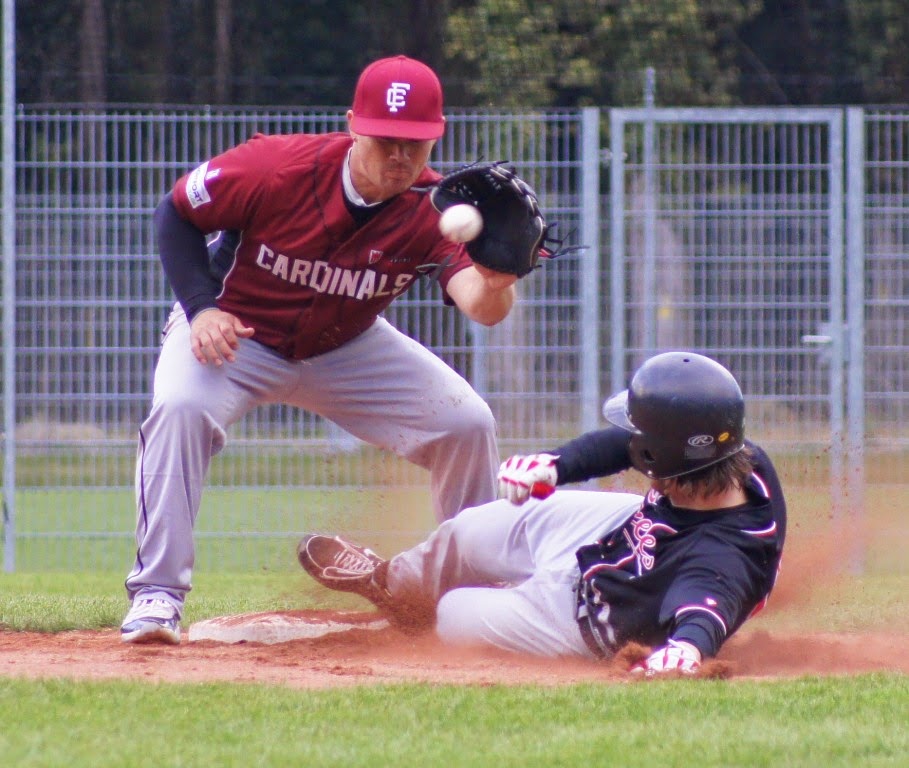The image captures a tense moment in a baseball game with a close-up of a play at either second or third base. A player in a dark blue shirt, white pants, and a blue helmet is shown sliding into the base, kicking up a cloud of dust and dirt. His white gloves with red details grip the ground as he slides. The base itself is covered with dirt from the action. The defender, wearing a red Cardinals jersey and a red baseball cap, is positioned behind the base, ready to catch the ball with his black mitt. The ball is just inches away from his glove. The defender's gray pants are slightly loose, and he is in a squatting posture, indicating the anticipation of the play. In the background, a silver metal fence and some trees are visible beyond the green grass and dirt of the field. Judging by the position of the sliding runner, it appears he might be safe as his foot is just about to touch the base.